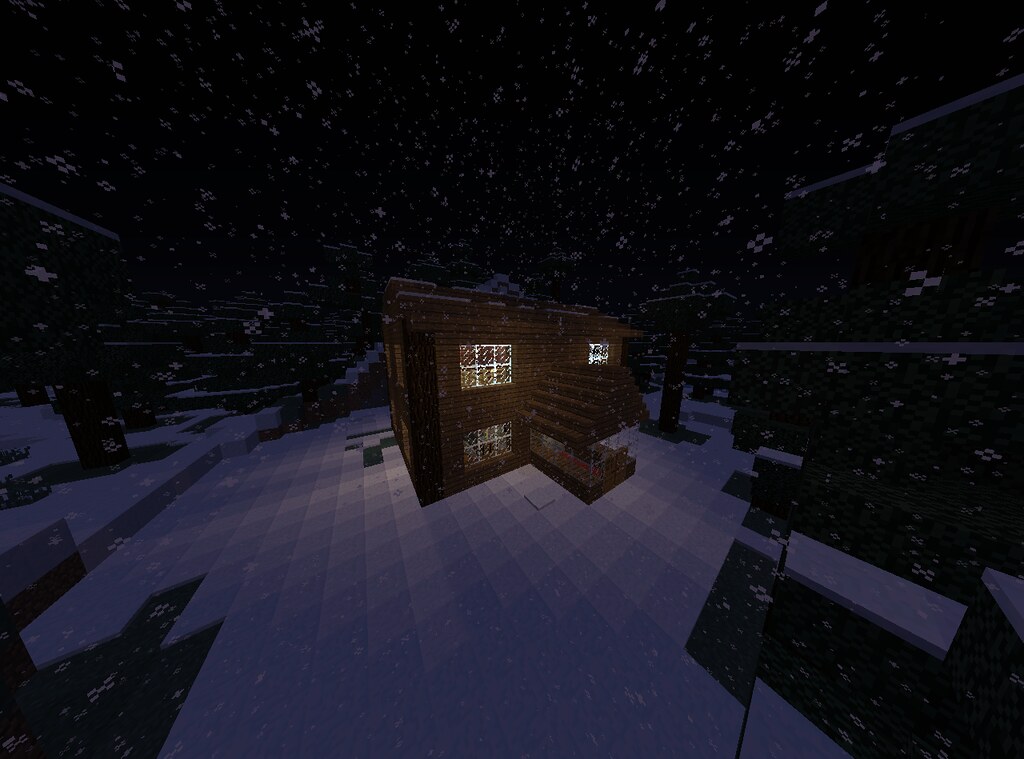This computer-generated image appears to be from a video game, showcasing a snowy scene with a pixelated, Minecraft-style aesthetic. Dominating the center of the image is a large, square, brown brick house, oriented slightly diagonally. The house features a prominent overhang or canopy extending over a porch area, and it has windows on both the top and bottom floors. Each of the four windows is divided into six panes by white frames, enhancing the pixelated theme.

The ground is depicted as a grid of white squares, representing snow in a tile-like pattern. To the left of the house, there is a section that hasn't been filled in with these white squares yet, adding to the digital nature of the scene. The sky is a solid black and is filled with tiny, diamond-shaped pixels falling like snowflakes from all directions, reinforcing the wintry atmosphere.

In addition to the house, a tree is visible to the right, and other similar boxy structures can be seen in the distance on the left. The entire scene is depicted in a highly stylized, pixelated manner, emphasizing the game's retro, digital design.